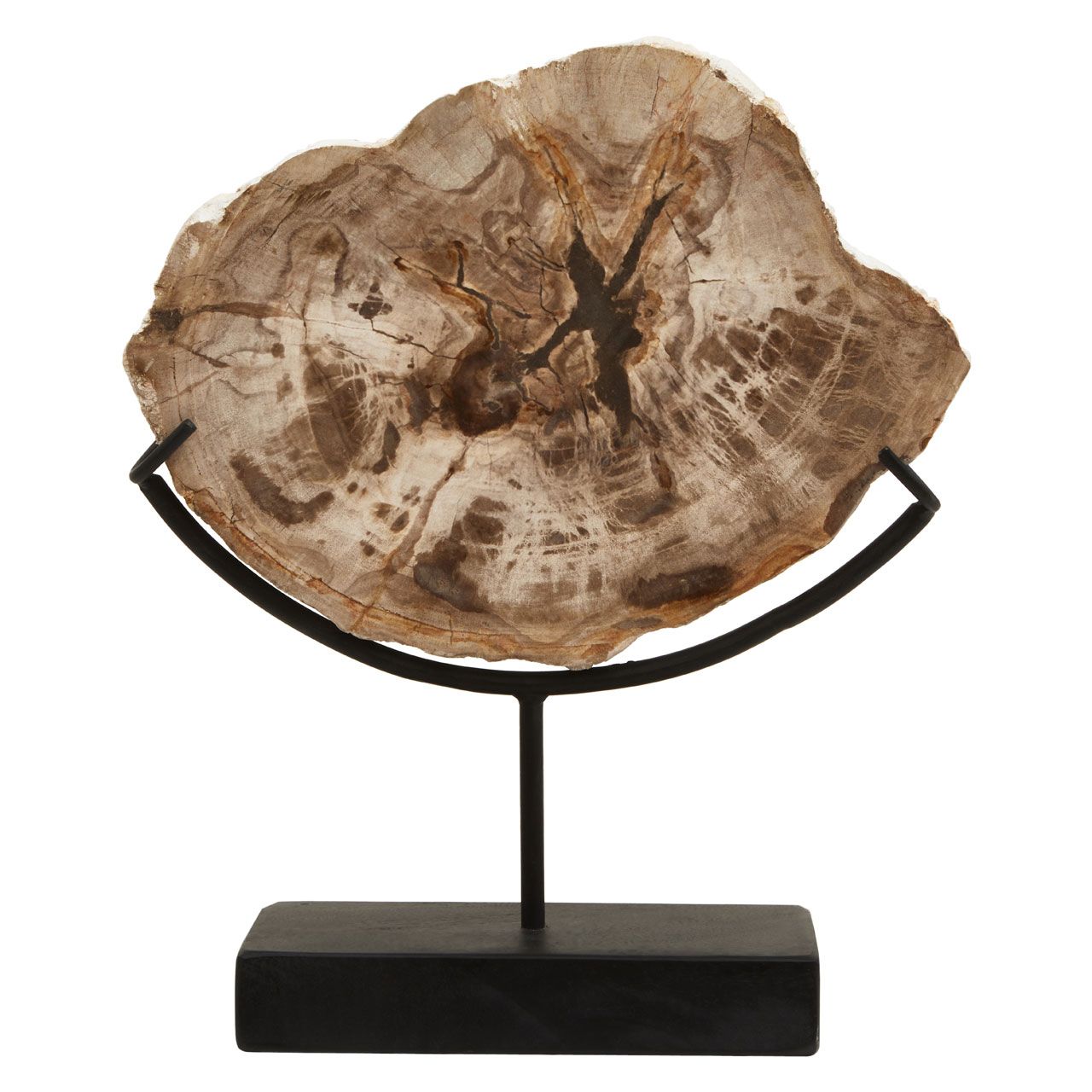The image features a detailed and artistic display with a pure white background. At the center, there’s a sizable, vertical cross-section slice of a tree, resembling a sliver or pancake cut from the trunk. The wood is prominently brown and dried with numerous visible veins and tree rings, indicating it may be from an old and possibly unhealthy tree given the dark knot at its core. The slice is mounted on a unique stand with a sturdy black rectangular base and a metal rod extending upwards. This rod connects to a rounded, curvy frame that holds the wood securely in place with two rounded hooks. The wood's varying hues range from light gray and white to various shades of brown, highlighting its aged and weathered texture. The meticulous display suggests it could either be a decorative piece or an exhibit in a museum.